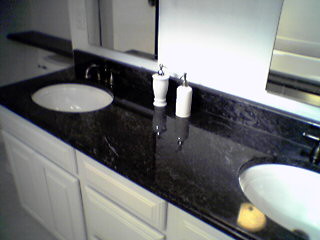This image showcases a luxurious double vanity bathroom setup. The countertop is crafted from striking black marble with delicate white veining, adding a touch of elegance to the space. The dual sinks feature pristine white basins complemented by dark metal-colored fixtures, enhancing the modern aesthetic. Centrally positioned between the sinks are two white soap dispensers, each topped with metal nozzles. Above each sink hangs a mirror, reflecting the white walls and creating a sense of spaciousness. The cabinetry beneath the sink is also white, providing a clean and cohesive look.

The highly-polished marble countertop reflects ambient lighting, which also casts a glow on the soap dispensers and the glistening sink surfaces. To the left of the vanity, part of the toilet tank is visible, capped with a flush mechanism, and adorned with a small shelf above it. Although only a small portion of the floor is shown, it appears to be light-colored, possibly white, contributing to the room's airy atmosphere. The mirrors reveal subtle glimpses of the bathroom's other side, maintaining the room's cohesive and sophisticated design.